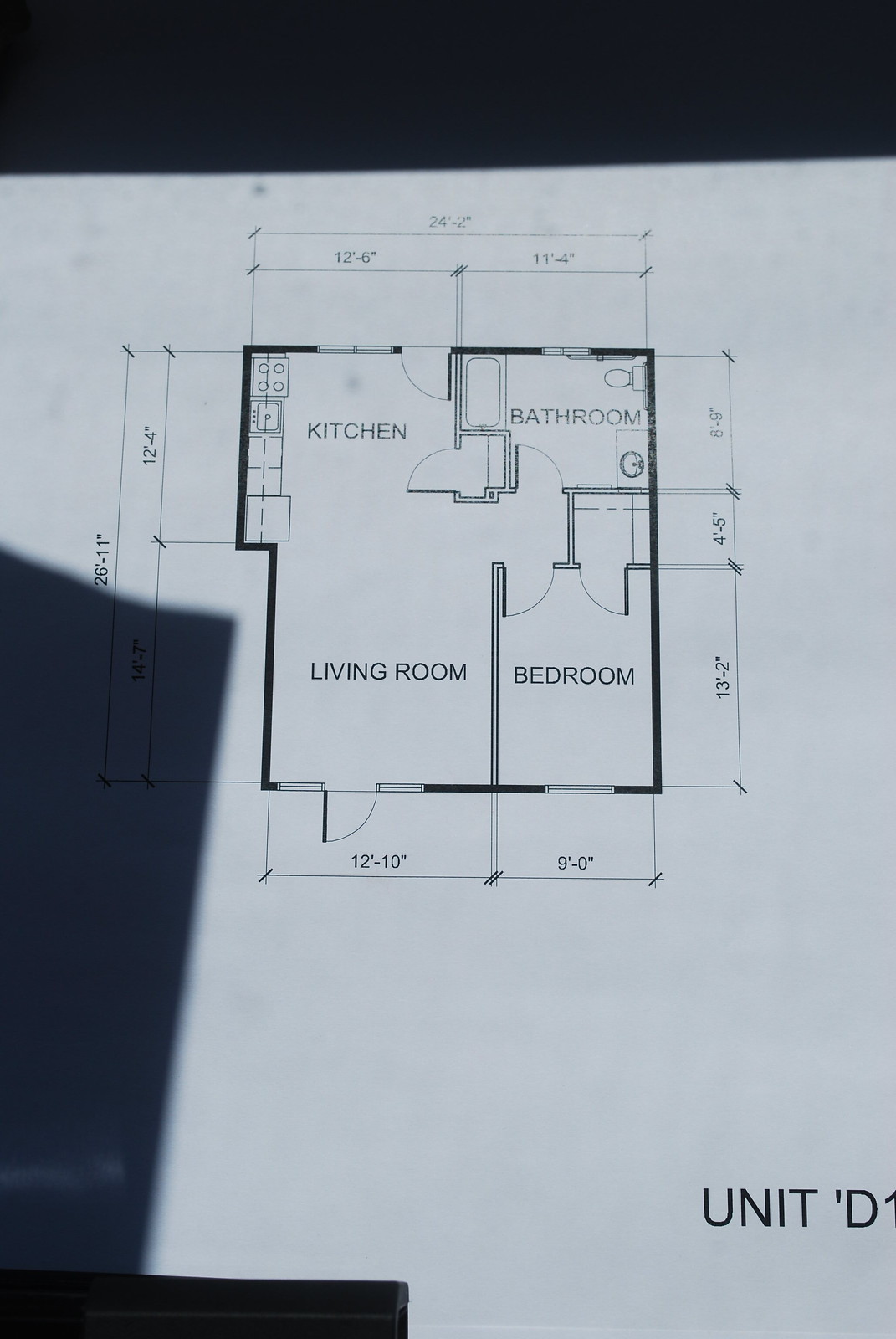This photograph depicts a detailed floor plan for an apartment designated as Unit D, showcased at the bottom right corner. The layout includes marked dimensions for each room and specific areas within the unit. Notable measurements are clearly labeled: the kitchen is 12 feet 6 inches, the bathroom measures 11 feet 4 inches, and adjacent to the kitchen is a section noted as 12 feet 4 inches. Although a shadow masks the dimension in front of the living room, the other dimensions are visible with the living room itself measuring 12 feet 10 inches and the bedroom at 9 feet 0 inches. The area to the right of the bedroom is 13 feet 2 inches. Additionally, next to the bathroom are two distinct spaces sized at 4 feet 5 inches and 8 feet 9 inches. The overall image orientation is taller than it is wide, with no individuals present in the photograph.